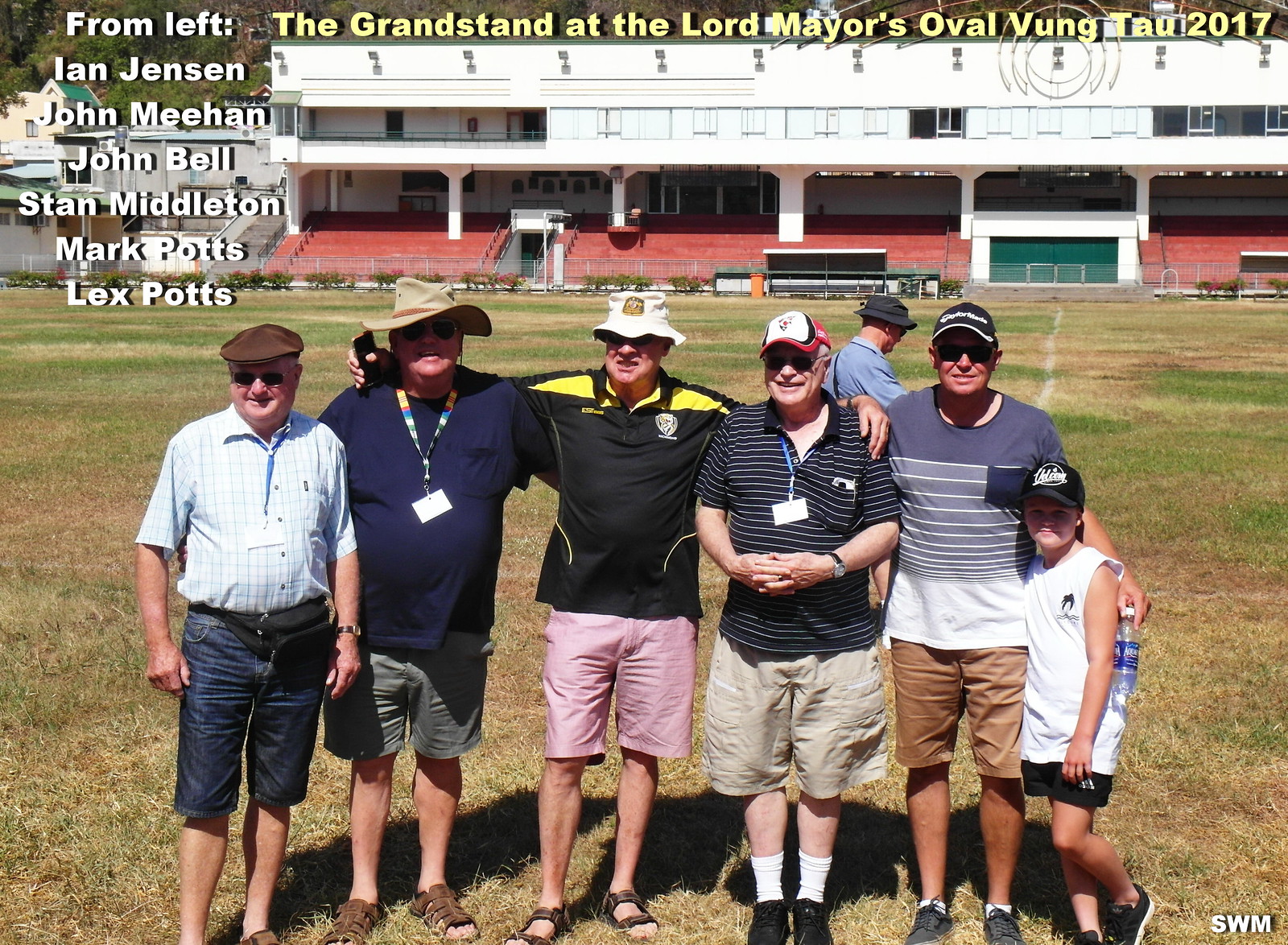This image captures a group of six men and a little boy standing and posing on a field, likely a football or soccer field, adjacent to red bleachers of a grandstand. They are all dressed in shorts and short-sleeved shirts, suggesting a warm day. The top of the image features yellow text reading, "The Grandstand at the Lord Mayor's Oval, Vung Tau 2017." Below this, white text identifies the group from left to right as Ian Jensen, John Meehan, John Bell, Stan Middleton, Mark Potts, and Lex Potts. The men stand on green and yellow grass with some brown and white lines indicative of the field's markings. Their attire includes a variety of hats, shirts, shorts, and shoes, with specific details such as a black fanny pack and distinctive hats and shirts mentioned for each individual. Behind them, there's a silver fence spanning the width of the image, and further in the background, white buildings with green roofs. A man in the background, who appears to be separated from the group, is facing away from the camera. The boy, positioned on the far right, is dressed in a black hat, a sleeveless white shirt, black shorts, and black and white shoes. The scene is lively, capturing a moment of camaraderie and possibly celebration or documentation at the sports venue.